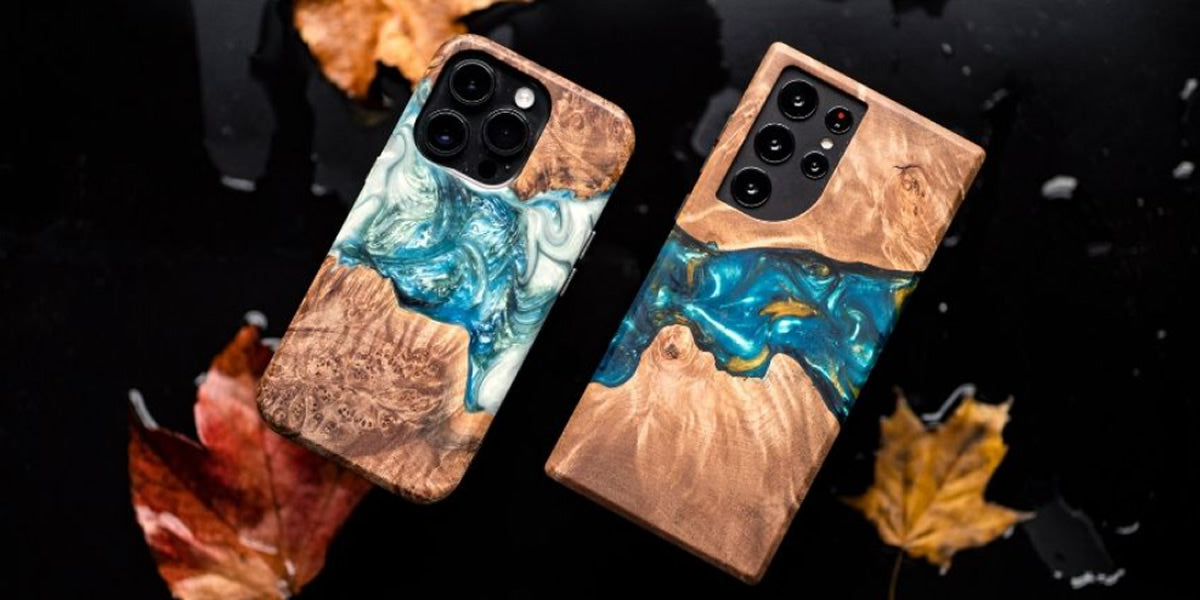This image features the back of two high-end cell phones, each in a casing with intricate designs. Both phones are positioned on a black table, with the one on the right slanted and featuring five camera lenses (three large and two small). The phone on the left is slightly lower with three camera lenses. The cases are adorned with a mix of brownish and goldish colors interspersed with a sea or water motif rendered in various shades of blue, including turquoise. The surface they rest on is partially wet and partially dry, adding to the visual complexity. Around the phones are three distinct leaves: a yellow leaf in the bottom right, a reddish-brown leaf in the bottom left, and another brownish leaf at the top. This setting merges natural elements with modern technology, encapsulating the phones in a visually appealing and mysterious environment.